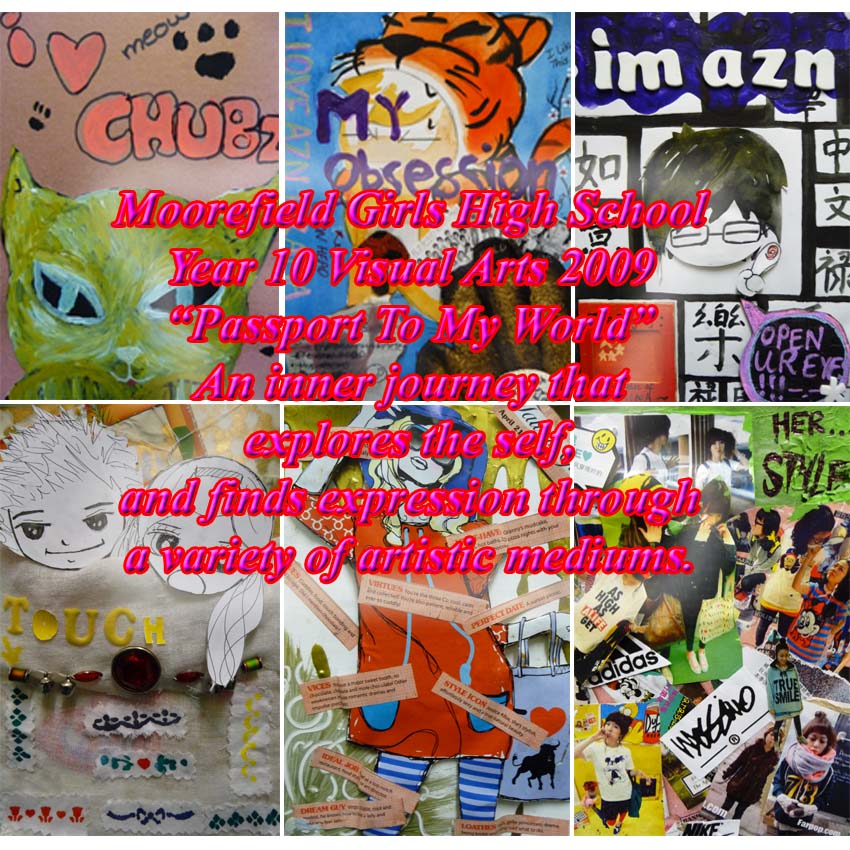This square image is a detailed digital collage divided into six equal sections, each showcasing a unique blend of cartoon-like drawings, newspaper clippings, and artistic text. 

In the top left corner, against a brown background, there's a green cat with black eyes and a white nose, surrounded by pink hearts and black paw prints, with the words "Meow" and "Chubs" (C-H-U-B-Z) painted in orange. 

The top center section features a vibrant blue background with a painting of a tiger, mouth open, accompanied by the text "my obsession." 

To the top right, a drawing of an Asian character with glasses is depicted with the phrase "I'm AZN," and around it are Japanese writing and the words "open your eye" within a purple circle.

Moving to the bottom row, the lower left corner shows the heads of a boy and girl drawn on white paper, with the word "touch" written in yellow beneath them, and adorned with small beads and patterned cloth underneath.

The bottom center section presents a colorful cartoon of a lady with long blonde hair, wearing sunglasses, a floppy blue hat, a red dress, and blue-striped pants, holding a bag with a red heart. Texts scattered around her include phrases like "vices" and "style icon."

In the bottom right corner, there are multiple images of people in various activities, paired with large texts such as "Adidas" and "her style."

Across the top and bottom rows in pink text with a red outline, the caption reads: "Moorfield Girls High School Year 10 Visual Arts Show 2009 'passport to my world' an inner journey that explores the self and finds expression through a variety of artistic mediums."